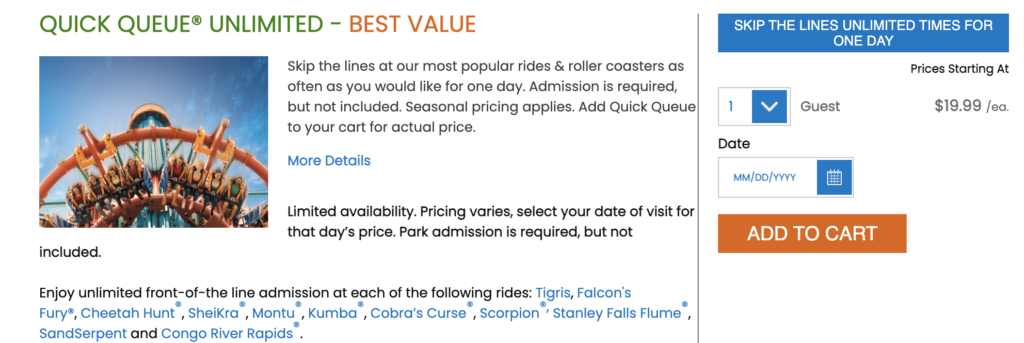The web page promotes a one-day, unlimited-use pass called "Quick Queue" for an amusement park, offering guests the convenience of skipping lines for the park's most popular rides and roller coasters. At the top of the page, a header announces "Quick Queue Unlimited Best Value." Below this, in black ink, additional information is provided: 

"Skip the lines at the most popular rides and roller coasters as often as you would like for one day. Admission is required but not included. Seasonal pricing applies. Add Quick Queue to your cart for the actual price."

A clickable tab labeled "More Details" reveals further information, detailing that availability is unlimited but pricing varies based on the selected visit date. The tab underscores that park admission is mandatory but not part of the Quick Queue purchase.

A vivid image of a thrilling vertical drop ride captures the excitement the pass offers. Beneath this image, text invites visitors to "enjoy front-of-the-line admission at each of the following rides," listing attractions in blue ink: Tigress, Falcon's Fury, Cheetah Hunt, SheiKra, Montu, and Kumba, among others.

To the right side of the page, a selection panel allows users to pick the pass. A blue button prompts with "Skip the lines, unlimited times for one day only," enabling the selection of the number of guests and visit date. Passes start at $19.99, with the exact price displayed after adding selections. An orange "Add to Cart" button is positioned below for finalizing the purchase.